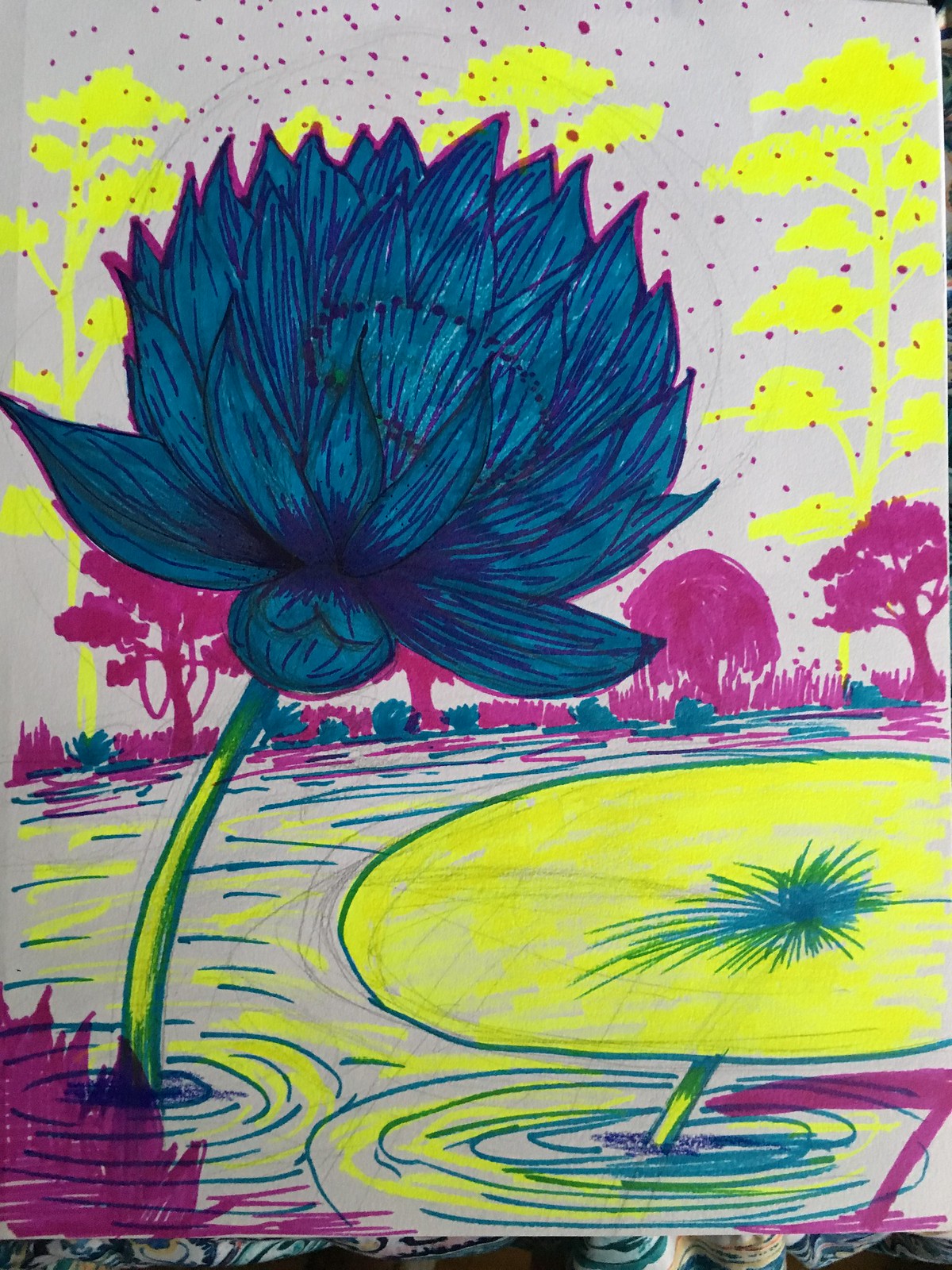The image showcases a vibrant blue flower with deep blue petals accented by light blue highlights. The petals are tall, long, and lush, densely grouped together. At the center of the flower, small, dark blue spheres form a striking focal point. The flower is supported by a green stem that transitions from a dark green base to a light, almost yellow hue, adorned with a prominent yellow streak. Attached to this stem is a large, flat yellow leaf, reminiscent of a lily pad, with green grass-like growth emerging from its top. 

Surrounding the flower are vividly colored trees, with some appearing in a rich magenta hue and others in a bright yellow, creating a dynamic and colorful backdrop. The plants in the foreground seem to rise from a body of water, depicted with lines of bluish-green and yellow that capture the wavy texture of the surface. This water is primarily the color of the page, an off-white, providing a neutral background that allows the vibrant colors of the flora to stand out dramatically.